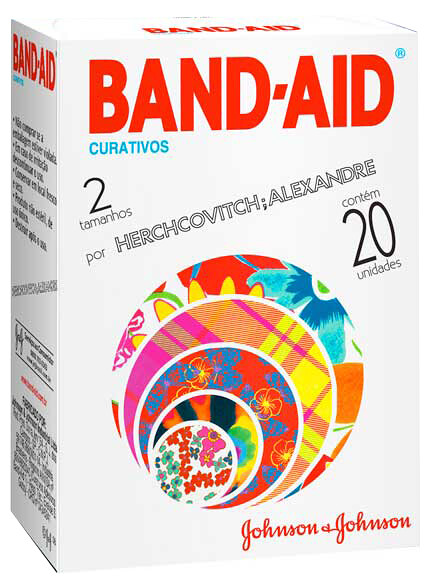The image is a close-up photograph of a Band-Aid box with no background. The classic white box features prominently the large red text "Band-Aid" at the top center of the closed lid, repeated on the left-hand side and the front. Below "Band-Aid," in light blue, it says "Curativos," which is the Spanish word for bandages. Further details in black and red text provide additional information in Spanish, including "dois tamanhos por Herchcovitch Alexandre" and "contem 20 unidades." The top right corner has an "R" with a circle around it in light blue, indicating a registered trademark. The bottom right corner of the box shows the red logo "Johnson & Johnson." Prominently featured on the front are concentric circles displaying different Band-Aid patterns, such as floral, plaid, and tiger stripes, each in bright, fun colors. This image effectively showcases the variety of decorative bandages available in the box.